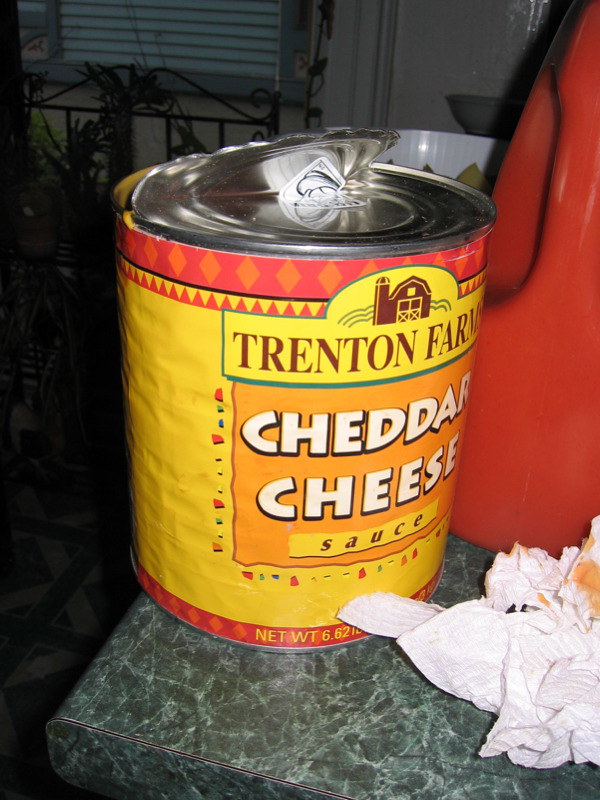The photograph captures a large metal can of cheddar cheese sauce partially opened, with the lid bent back by a can opener, revealing the contents inside. The can has a predominantly yellow label with red and orange bands at both the top and bottom edges and features a picture of a barn with the brand name "Trenton Farms" depicted in brown letters. The label also prominently displays "Cheddar Cheese" in white letters and "Sauce" in black letters. The can is situated on a green marbled Formica countertop. Beside it lies a crumpled white paper towel with traces of the orange cheese sauce and a red plastic bottle, likely containing ketchup or salsa. Additionally, a gallon-sized orange jug is partially visible in the background, and there is a window showing a black wrought iron fence beyond the countertop.